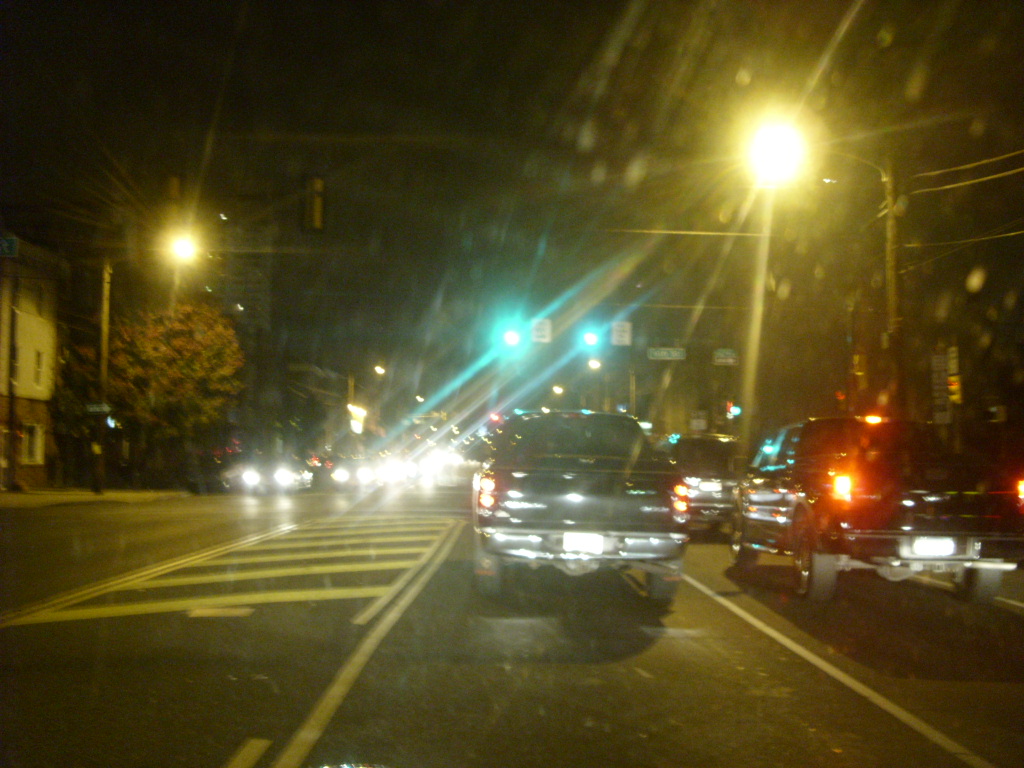This nighttime photograph is taken from the inside of a car, likely from the front passenger seat, as it approaches a green-lit intersection. The windshield is dirty, causing the numerous streetlights, traffic lights, car headlights, and taillights to create a streaky, blurred effect, reminiscent of simulated astigmatism. Directly ahead and to the right are two black pickup trucks, while to the left, the oncoming traffic lane reveals bright headlights. The scene is set in an urban, semi-residential area lined with low-rise apartment buildings and commercial structures. The street, which includes a turning lane in the center, has freshly painted yellow lines. A strong street light in the top right corner reflects heavily off the grime on the windshield. The traffic seems dense, with vehicles slowly starting to move as the light has recently turned green.